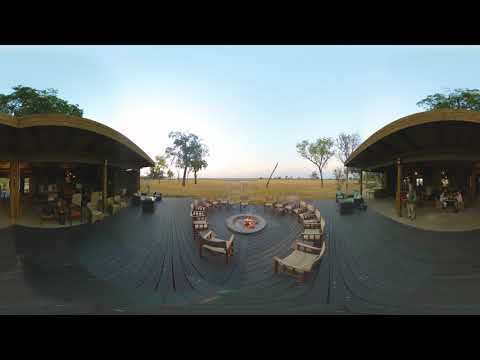The image captures an expansive outdoor scene with a wide-angle lens that distorts the spatial characteristics. In the foreground, there is a communal seating area featuring a circle of wooden chairs surrounding a campfire or fountain. On either side of the seating area stand two small structures, possibly huts or buildings, that might serve as homes or stores; their interiors remain obscured by darkness. People are seen milling about inside these buildings, although their activities are unclear. There are several cars parked in front of both structures. The setting seems quite ceremonial, as if prepared for a wedding, with prominent seats in the forefront perhaps reserved for the couple and an officiant. The fire already lit adds to the ceremonial vibe. The background features an open field dotted with a few small, young trees. Above, the sky is mostly clear with hints of white, tent-like formations that could be interpreted as light clouds. One solitary figure stands near the seating area, conveying a sense of solitude against the backdrop of an otherwise anticipatory scene.